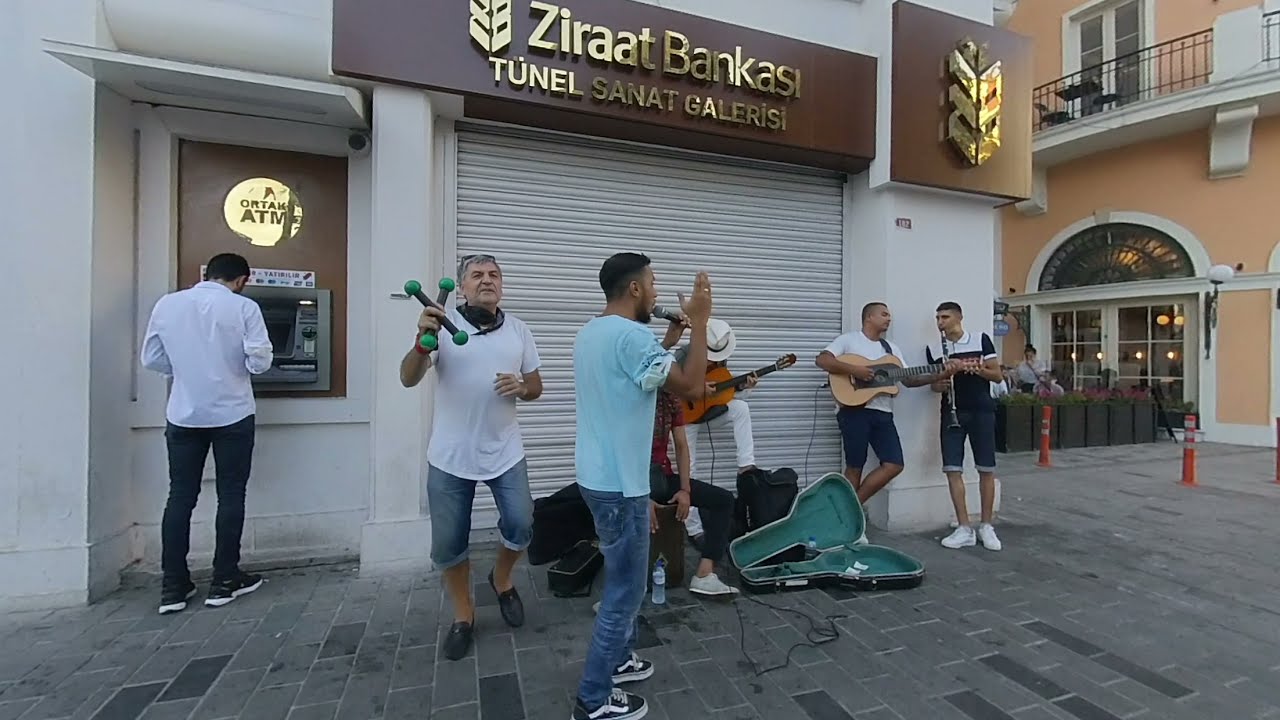This detailed photograph captures a lively street scene featuring a group of buskers performing in a town square. The performers, including two guitarists, a flutist, a man with a microphone, and another with an unusual instrument with green knobs, are positioned in front of a white building. The building is identified as "Zirat Bankski Tunnel Sanat Galerisi" by the golden text on a brown sign above a closed shutter. To the left of the band, a person is seen withdrawing money from an ATM, while to the right, a brown-walled building is visible. The ground is paved with gray rectangular bricks. Additional details include a musician playing a bright orange guitar and a glimpse of an outdoor dining patio nearby, where people are seated, adding to the street's bustling atmosphere.